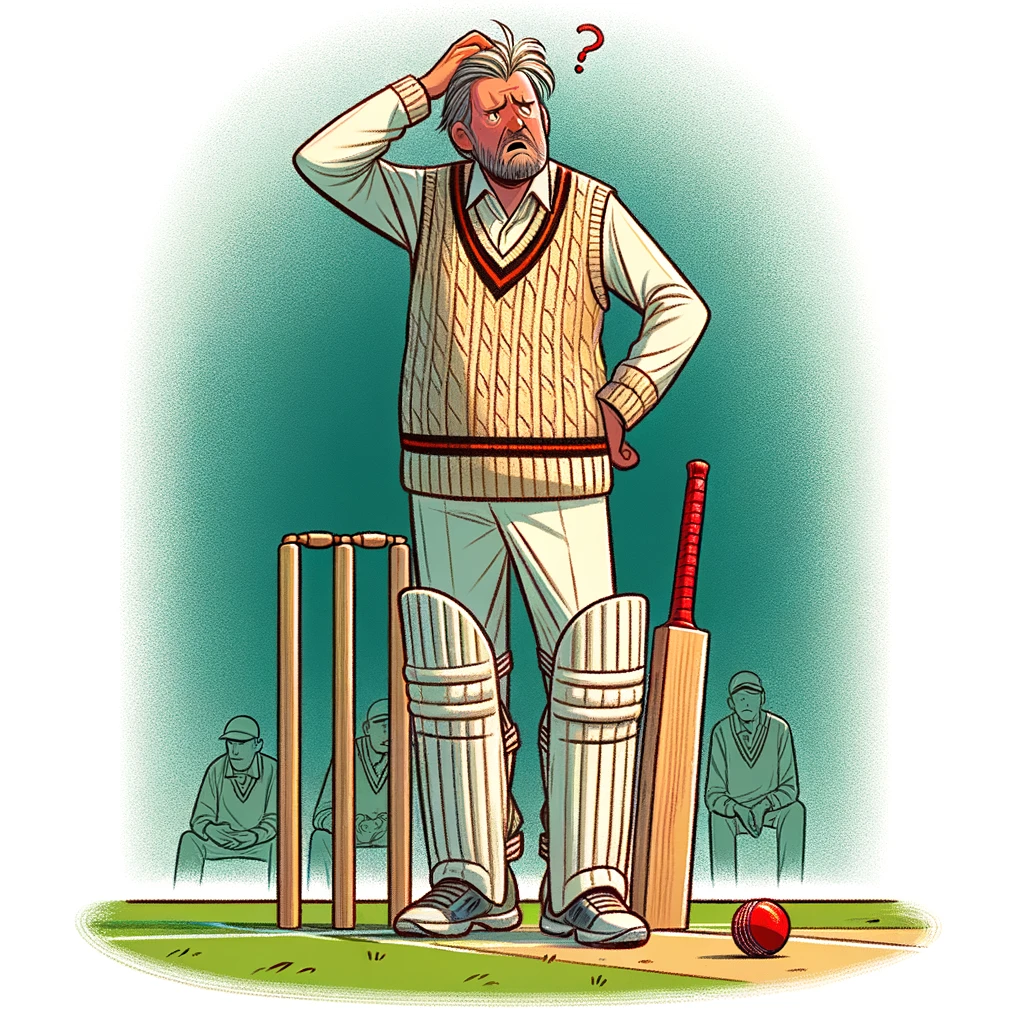This is a cartoon image showcasing an older man with long gray hair, scratching his head with a puzzled expression. He is standing in the forefront, wearing a white long-sleeved collared shirt, a sweater vest with red and black ribbed stripes at the neckline and bottom, white pants, shin guards, and white tennis shoes. A red question mark floats above his head, emphasizing his confusion. The scene appears sports-related, possibly cricket, as there are three wickets to the left and a cricket bat with a red handle on the right. A red ball lies near the bat. In the background against an aqua blue sky, three silhouetted figures in similar uniforms are seated on a bench, adding to the overall cricket theme. The grass, a bright green, complements the vibrant setting of this comic-like drawing.